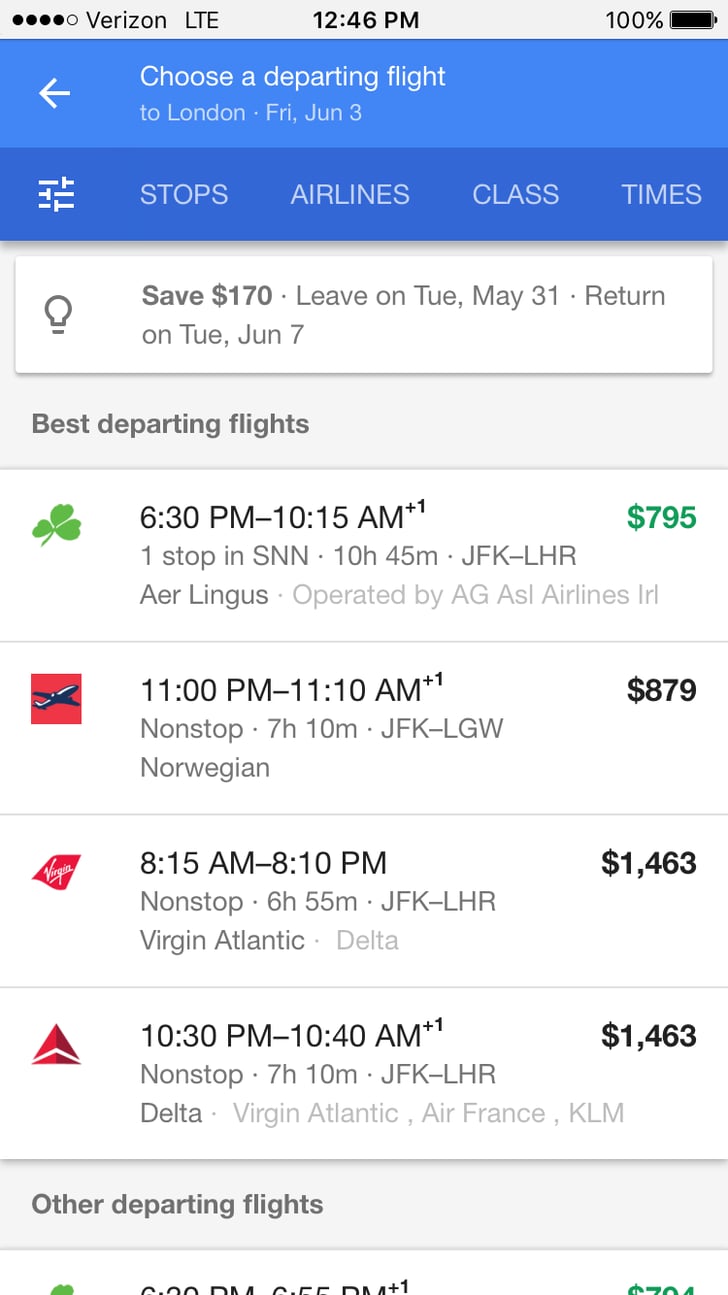This detailed caption is for a screenshot of a phone displaying a flight search result screen:

The screenshot captures a flight search result screen on a mobile device. At the very top, there's a thin gray border. In the top left corner, five small black circles are aligned horizontally next to a gray circle with a black border. To the right of this, the word "Verizon" appears in black, followed by "LTE" in all capitals. At the center of the top border, the current time is displayed. Towards the right, there is a battery icon to the left of which reads "100%."

Just below this top border is a blue section that houses a white left-pointing arrow in the center-left. Next to the arrow, white text reads "Choose a departing flight." Underneath this, in smaller font, it says "To London - FRI, June 3rd."

Moving down, there is a slightly darker blue bar, which contains three white lines with small notches on the far left. To the right of these lines, in white capital letters moving left to right, are the words: "STOPS," "AIRLINES," "CLASS," and "TIMES."

Beneath this, a white rectangle includes a light bulb icon on the left side. To the right of the icon, bolded black text says "Save $170," followed by plain black text: "Leave on Tuesday May 31st. Return on Tuesday, June 7th." Below, a light blue border contains bolded black text stating "Best Departing Flights."

Within this section, there are four listed flights, each separated by a thin light gray line. Each entry shows the flight company's icon on the left, the departure time, number of stops (non-stop, one stop, etc.), layover duration, and airline name in the center, with the price displayed on the right.

Further down, another thin light gray line separates this section from the next, where black text on the left side reads "Other Departing Flights." Below this is a white border, with the partial top of some text cut off at the bottom of the screen.